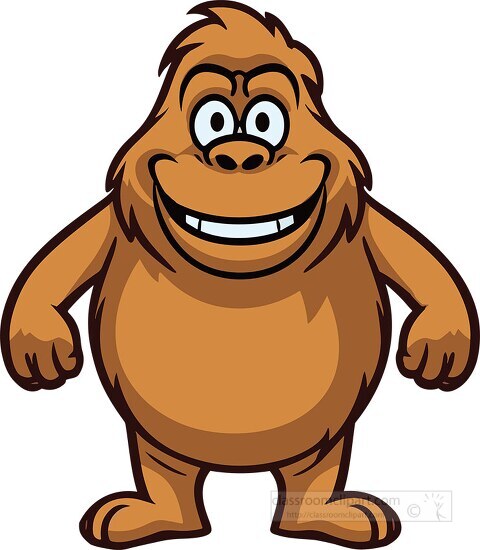This is an animated image of a very happy-looking gorilla, positioned against a solid white background with no borders. The gorilla, outlined in thick black lines, is facing the viewer with large, expressive white eyes and oval black centers. Its short legs support a very round, almost circular stomach area, with arms held out wide and fists facing forward. The gorilla's mouth curves upward into a big smile, revealing a rectangular white center with two smaller rectangles on each side for teeth. It has feathery dark brown fur, accented with some light brown touches, particularly noticeable on top of its head and around its cheeks. The whole figure exudes a cheerful, cartoonish charm.